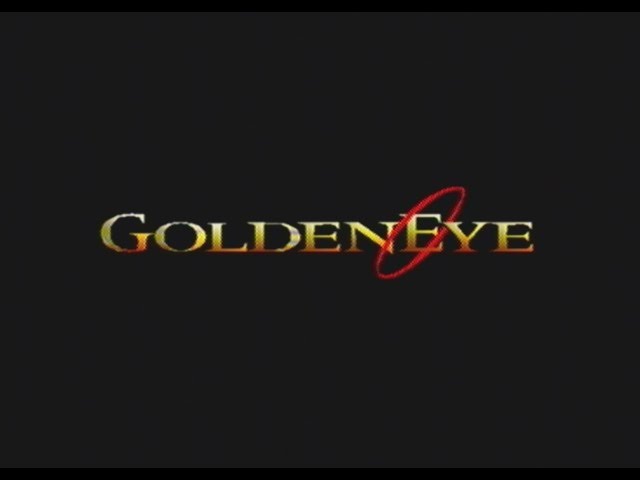This image is a screenshot possibly taken from a computer screen, depicting what appears to be the logo for the James Bond franchise "GoldenEye 007," a video game. The background is completely black, creating a stark contrast with the bold, gradient-colored text "GoldenEye," which progresses from a white hue at the top to a deep orange at the bottom, giving it a golden appearance. The font is classic and uniform, with all characters in capital letters. A distinctive red oval is circled around the first "E" and the "I" in "GoldenEye," adding a stylized touch to the design. The red oval slightly intersects with the 'N' and protrudes below the upper left corner of the 'Y,' further integrating into the logo's composition. The overall image is slightly blurry, indicative of its origins as a screenshot, possibly enhancing its vintage video game aesthetic.